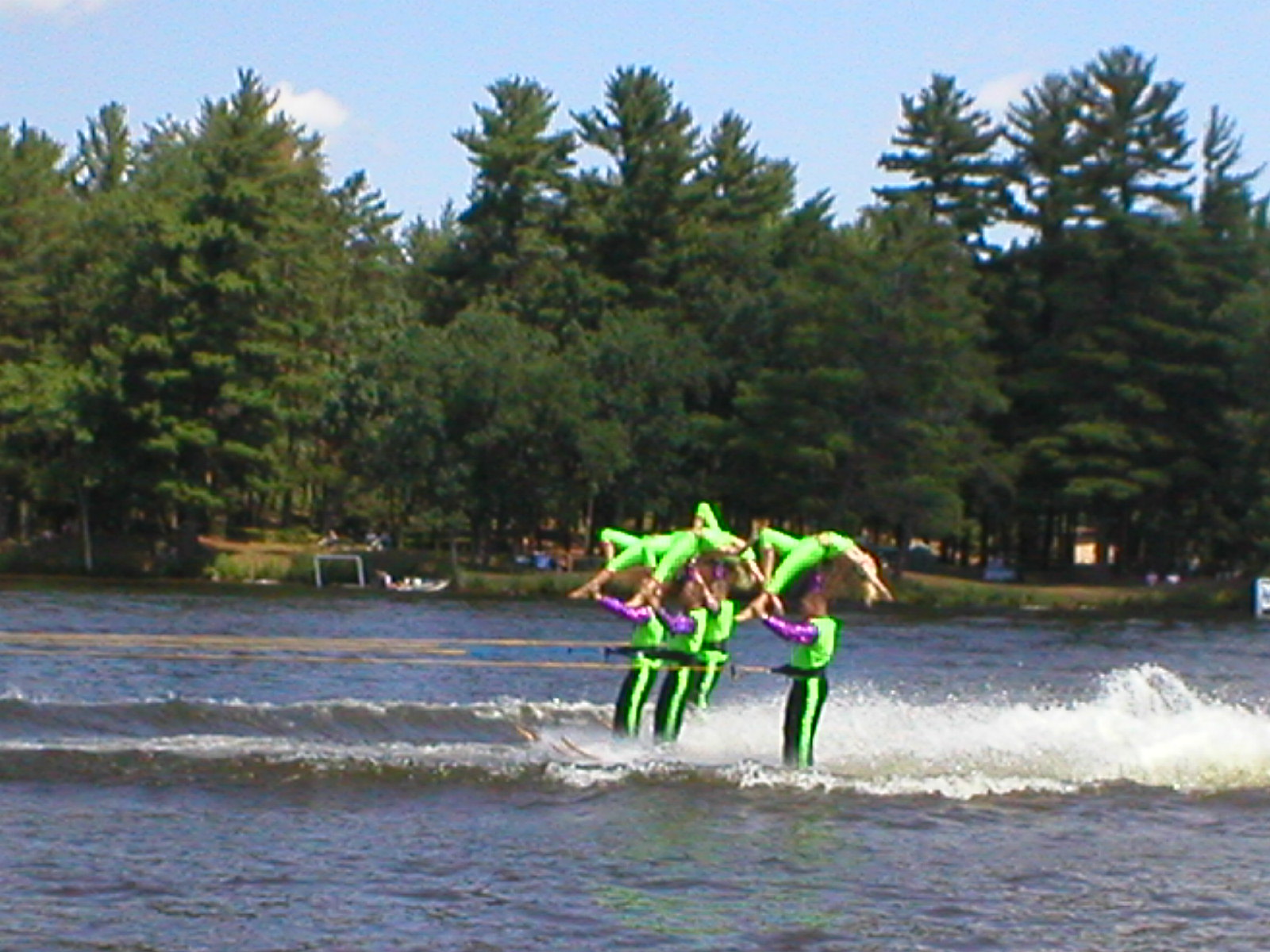The photograph captures a vibrant and dynamic scene of four men engaged in water skiing on a lake, seamlessly blending the thrill of the sport with an impressive display of balance and coordination. The men, clad in shiny purple long-sleeve shirts paired with green vests and black pants featuring a bright green stripe, are shown being pulled by a boat, with the tow ropes visibly secured around their waists. Each man is skillfully balancing a woman over his head; the women are dressed in matching outfits with bright green pants and tank tops. They pose elegantly with their backs arched, hair flowing backwards, and one knee bent, adding a touch of grace to the athletic spectacle. The skis carve through the water, creating waves and a wake behind them. The backdrop is a picturesque landscape of tall fir and pine trees lining the bank of the lake, under a clear blue sky, enhancing the serene yet exhilarating atmosphere of the image.